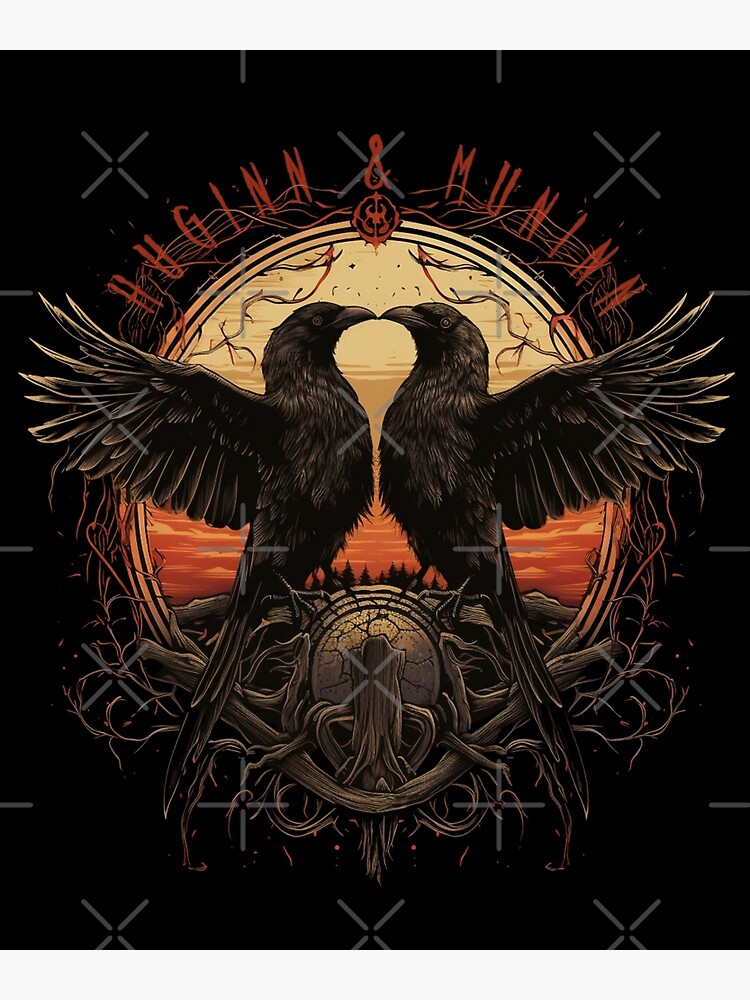The image features a vertical rectangular design set against a very dark, almost black, background. Dominating the composition are two black birds, likely crows or ravens, crafted from metal. The birds face each other with their beaks touching and wings spread apart, creating a striking and symmetrical display. They are perched atop what appears to be a coat of arms, also made of metal, and framed by twisted twigs or wooden logs.

Above and flanking the birds are intricate, darkened vines that add a decorative touch to the image. At the top of the design, in red letters, are the names "Huginn" and "Muninn," likely referencing Norse mythology. These names are separated by a small symbol. Below this text is an oval section resembling a painted window that depicts a sunset scene, featuring a light pale yellow fading into vibrant orange, with silhouettes of trees at the horizon. 

The entire image is overlaid with a watermark consisting of light gray X’s and crosses, which run across the picture to prevent unauthorized use. This detailed and darkly elegant image exudes a sense of mystique and mythological depth.